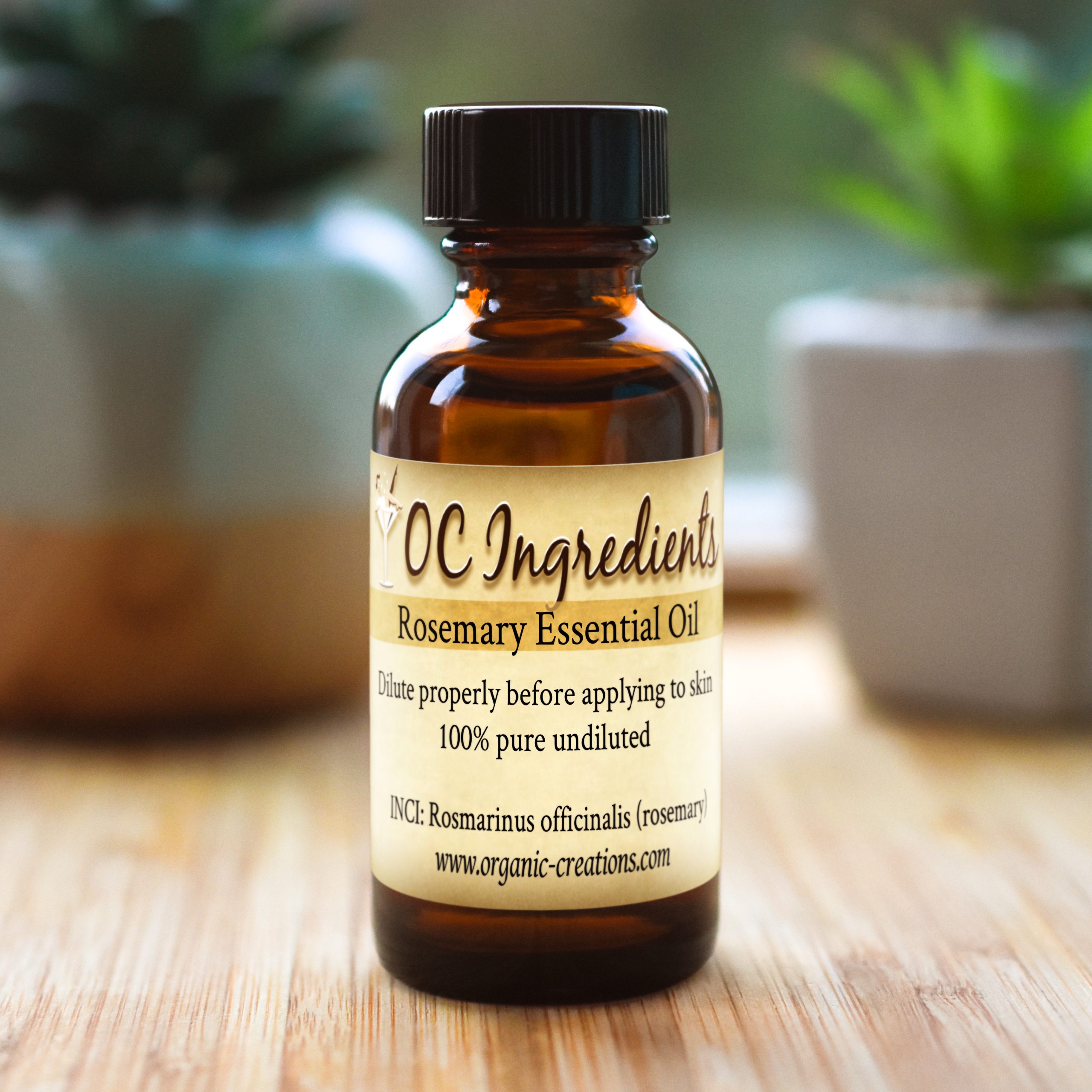This close-up, perfectly square photograph showcases a small brown glass bottle with a black plastic screw-on cap. The bottle features a tan-colored label with black cursive font that reads "OC Ingredients" at the top, followed by "Rosemary Essential Oil." Below, in smaller text, it states, "Dilute Properly Before Applying to Skin," "100% Pure Undiluted," and "INCI Rosmarinus Officinalis Rosemary." The web address "www.organiccreations.com" is printed at the bottom. The bottle sits on a light tan wooden surface, and out-of-focus in the background are two potted plants. The plant pot on the right is solid gray, containing a small green leafy plant, while the one on the left is teal on top and brown at the bottom, with a darker green plant growing from it. The image sharply focuses on the bottle, making the label and bottle details clear and prominent against the blurred background.